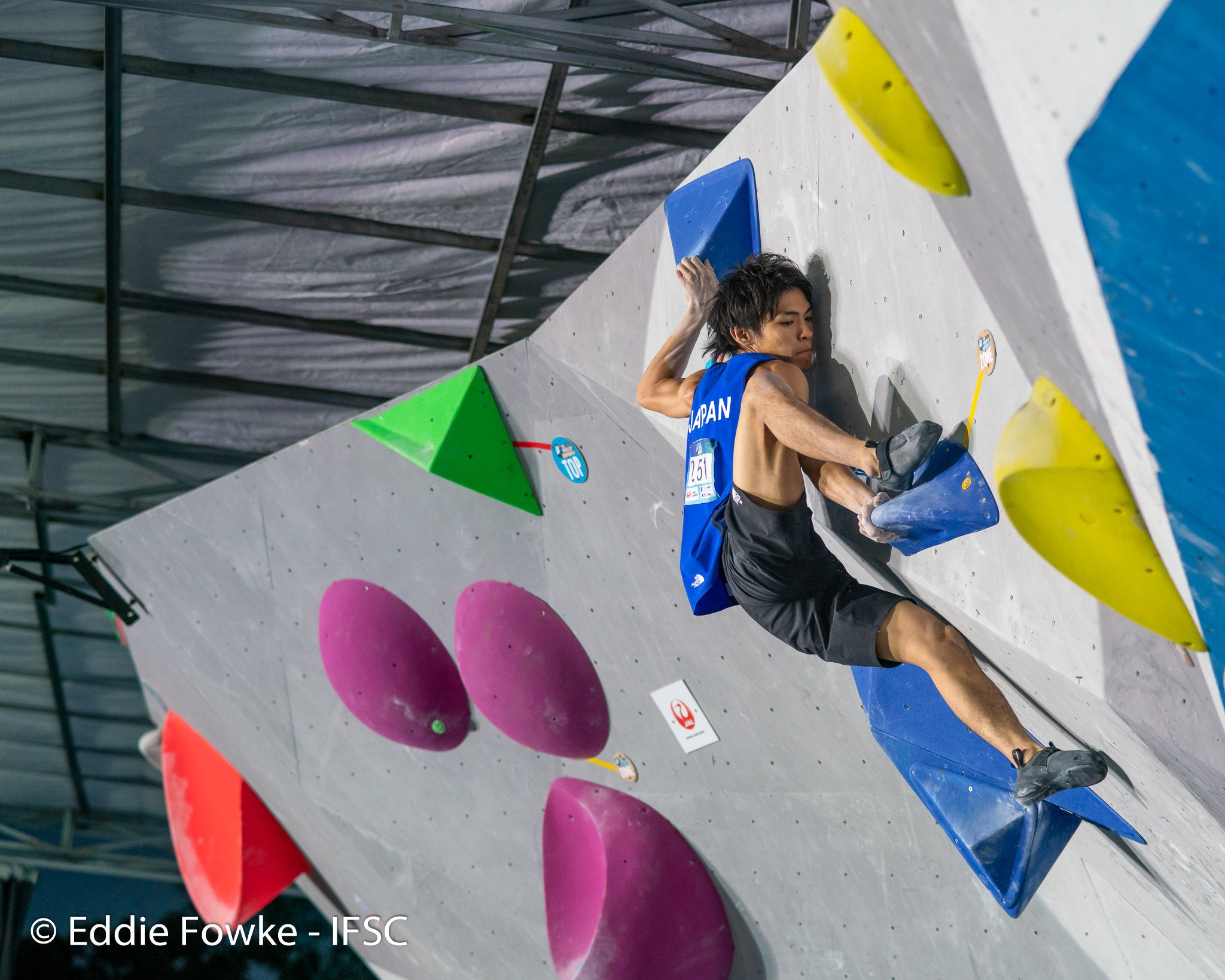This color photograph captures an intense moment of a competitive climber, identified by the number "251" on his blue jersey, scaling an indoor climbing wall. He appears to be an Asian man, showcasing his pronounced muscles and expert climbing skills, suggesting significant experience. He is clad in black shorts, gray climbing shoes, and a blue vest, with a white "Japan" emblem on it, indicating participation in a high-level competition. The climber's hands, dusted with white chalk, grip large, colorful handholds – notably three purple, three blue, one red, one green, and two yellow – which are disproportionately large compared to the usual climbing wall holds.

The wall itself is structured with a series of vibrant holds attached to a solid gray surface within the facility, designed to challenge climbers. The photo captures the climber's dynamic pose as he strategically places his right foot on a blue handhold, aiming to ascend higher. The white backdrop contrasts sharply with the lively colored footholds. Over to the upper left, a wrought iron structure and a gray curtain add depth to the scene, while the background hints at a professional setting without any visible ropes for safety, emphasizing the climber's confidence and expertise. 

The photographer's credit, "Eddie Fowke, IFSC," is prominently featured at the bottom left of the image, highlighting the prestigious international competition – the International Federation of Sport Climbing.